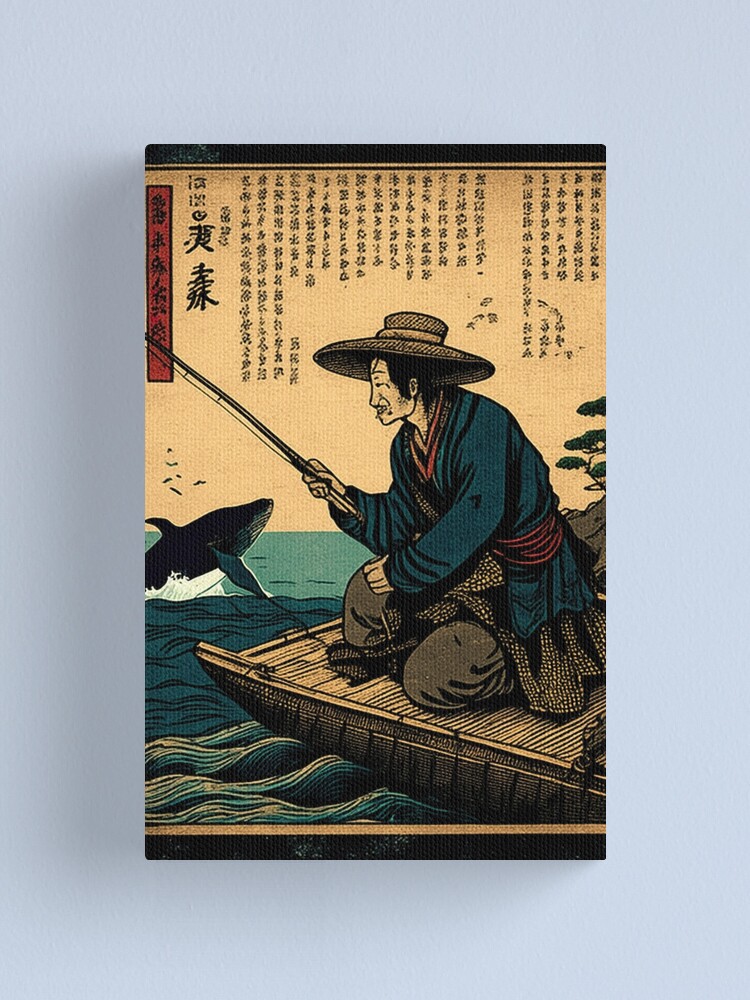The image is a vertically-oriented photograph depicting an ancient Asian scroll, set against a light blue or periwinkle background. The scroll itself has a manila parchment color with black borders at the top and bottom, possibly made of fabric. At the top of the scroll, there's Asian, likely Chinese or Japanese, text written vertically. In the center of the scroll is an elderly man, dressed in a flowing bluish-green kimono with a red scarf and black-and-white dotted tunic, paired with black pants. He is wearing a wide-brimmed straw hat. The man is fishing with a pole from a wooden dock, surrounded by water that appears to be the ocean. To the left of the man, a whale is seen leaping from the water, while on the right, branches of a tree, possibly a bonsai, are visible. The detailed and culturally rich imagery suggests that this piece would be fitting for a museum or for someone with a deep appreciation for Asian culture.